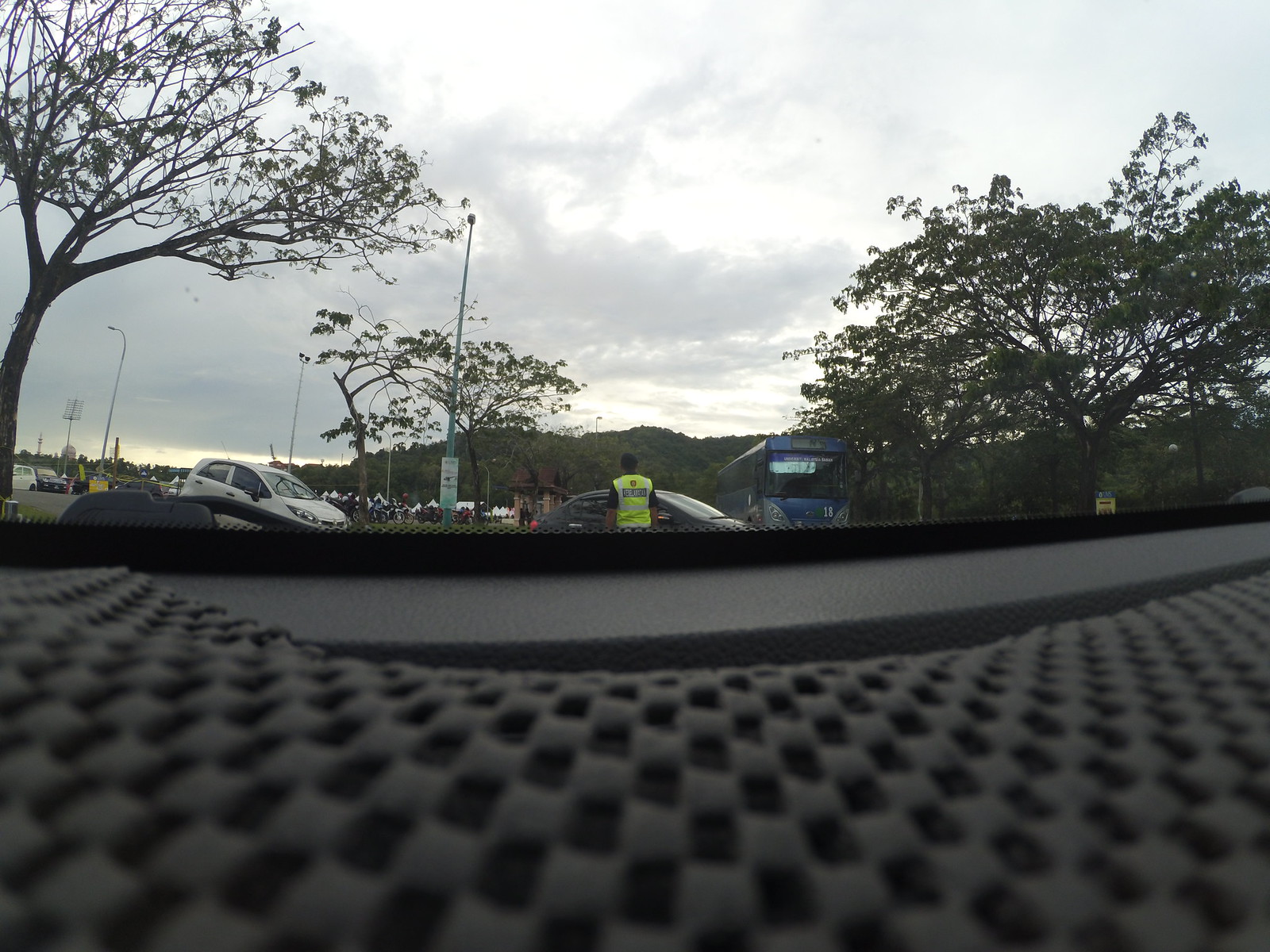Captured from an extremely low vantage point, this photograph prominently features a dark, perforated surface with a distinct checkerboard pattern in the foreground. Just beyond this textured surface stands a gray and black barrier which separates the foreground from the parking lot behind it. In the parking lot, several cars are neatly arranged, including a noticeable white car and a black car. Beside the black car, a man can be seen wearing a bright yellow safety vest, possibly engaged in some task. The background is marked by a line of trees on the horizon, with additional trees scattered throughout the parking lot, adding a touch of greenery to the scene.